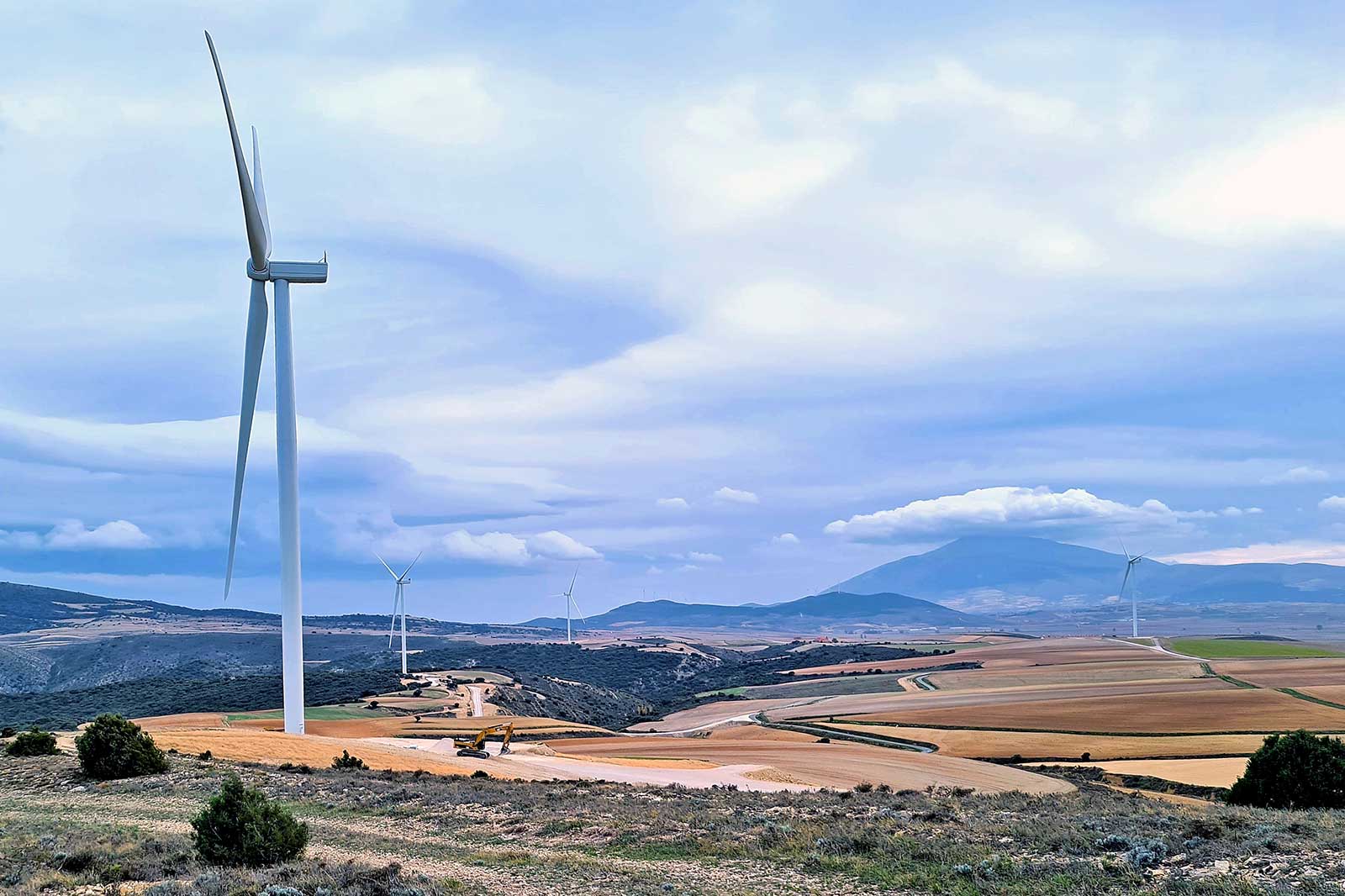The image portrays a vast, expansive outdoor landscape under a light blue cloudy sky, transitioning into darker hues as it moves downward. The foreground features patches of yellowish-brown dirt interspersed with occasional bushes and scattered patches of grass. As the eye moves further into the scene, the land stretches out into fields of similar yellowish-brown tones, which appear barren and desolate. Dotting this seemingly agricultural expanse are several large windmills, suggesting a wind farm presence. The mid-ground sees valleys and hills, some shrouded in bluish fog that adds a slightly mysterious ambiance. In the far background, blurred and faintly grayed-out mountains create a sense of depth, their peaks partially obscured by clouds. The entire scene evokes a serene yet somewhat deserted feeling, reminiscent of a semi-arid or desert-like environment with scarce vegetation and dominated by industrious windmills.